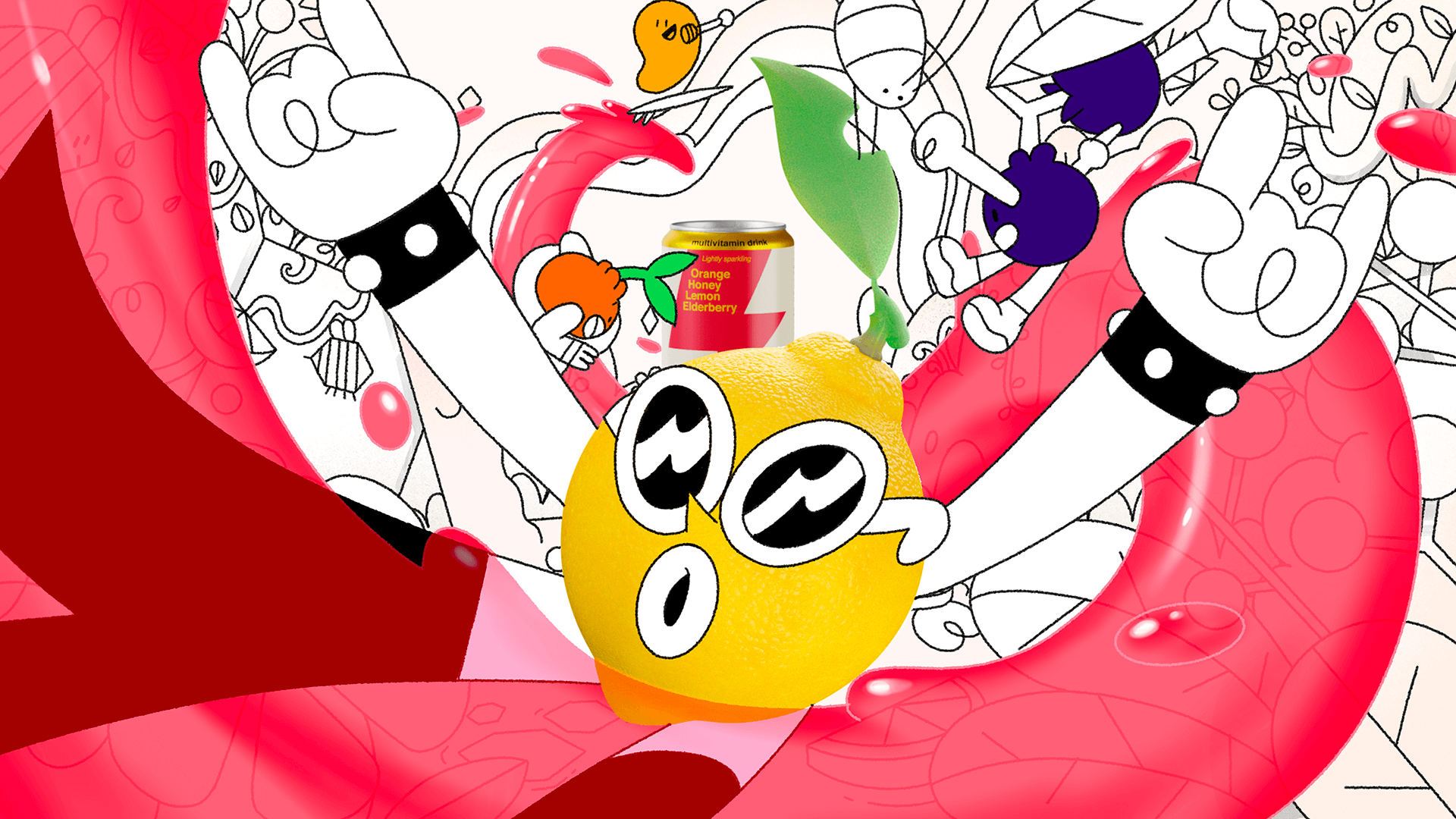The image is a vivid and dynamic cartoon advertisement for Rocket Panda Motion Graphics and Animation Studio. At the center, amidst a white background, is a yellow, lemon-like character with expressive eyes featuring black eyelids, a prominent white nose with black nostrils, and an 'O'-shaped mouth. Adorned with a small green leaf on top, the character is depicted in mid-gesture, arms extended, making a peace sign with both hands. The hands wear black wristbands dotted with white spots.

Surrounding this central figure is a riot of colorful, energetic elements: to the left, a swirling pink and red ribbon swoops under the character, encircling it and leading into the right side of the image where it reappears larger. Behind the main character, the chaotic background comes alive with various doodles and graffiti-like drawings. There's a pink and white pop can, purple-colored elements, a green fish, and a red balloon. Among these are also whimsical figures like bunny rabbits, ladybugs, a blue, long-necked ostrich-like creature, and several abstract shapes and squiggles. This collage of vibrant imagery creates a sense of motion and excitement, emphasizing the studio's creative focus.